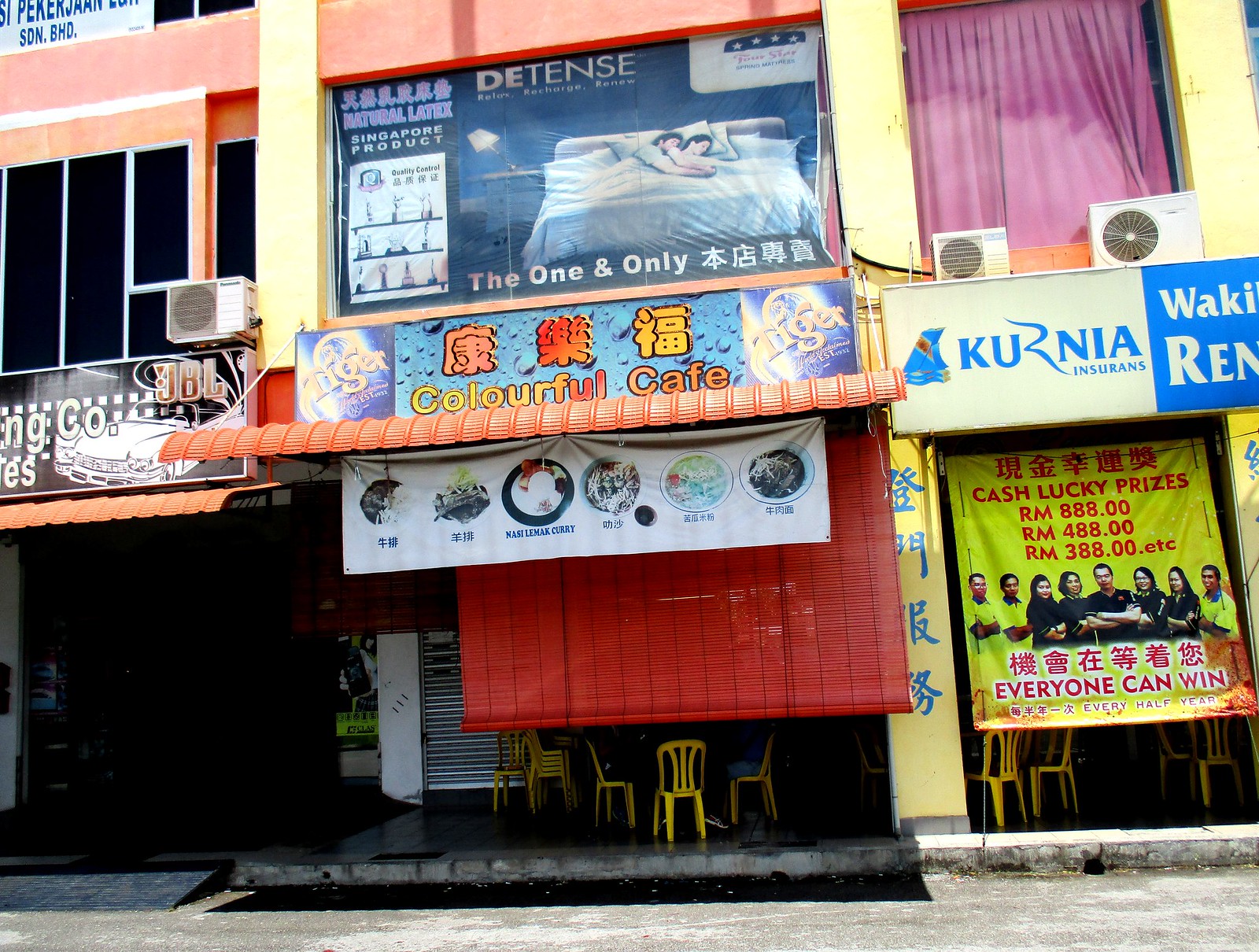This image captures an outdoor urban setting that appears to be in an Asian town, characterized by vividly colored storefronts and signage. Dominating the center of the scene is "The Colorful Cafe," prominently marked by a banner that reads its name. This cafe, easily identifiable by its yellow plastic chairs both inside and stacked, is currently closed, and various chairs are visible through large windows. To the right of the cafe is Kurnia Insurance, distinguishable by a blue and white sign. This store features decorative elements, including two fans and a pink curtain above the sign, with a yellow banner underneath that touts "Cash Lucky Prizes" with various amounts in RM (Ringgit Malaysia) like RM888, RM488, and RM388, promising everyone a chance to win every half year. On the left side of the image is a third storefront with blacked-out windows, an orange awning, and a black sign. Across the stone road, a curb delineates the edge of the walkway, contributing to the overall ambiance of bustling local commerce amidst colorful architectural elements, with hues ranging from tan and dark blue to lime green, pink, and purple. The entire setting is illuminated by daylight, enhancing the vibrancy of the different colored buildings accentuated in yellows, oranges, and reds.